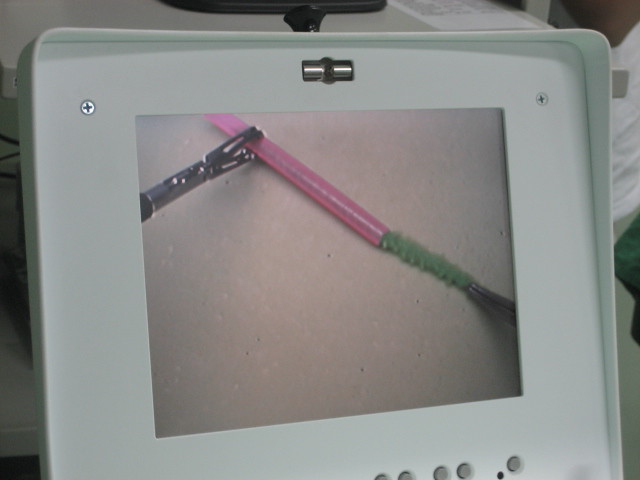This image depicts a close-up view on a screen, possibly captured using a microscope. The dominant element is a pink, straw-like tube, which appears to be a biological structure. Emerging from or entering this tube is a green, fuzzy object resembling a pipe cleaner in texture. The backdrop of the image does not provide any contextual details, leaving the focus entirely on the interaction between these two components. The coloration and texture hints at a possibly cellular or tissue-based scene, emphasizing the microscopic nature of the observation.